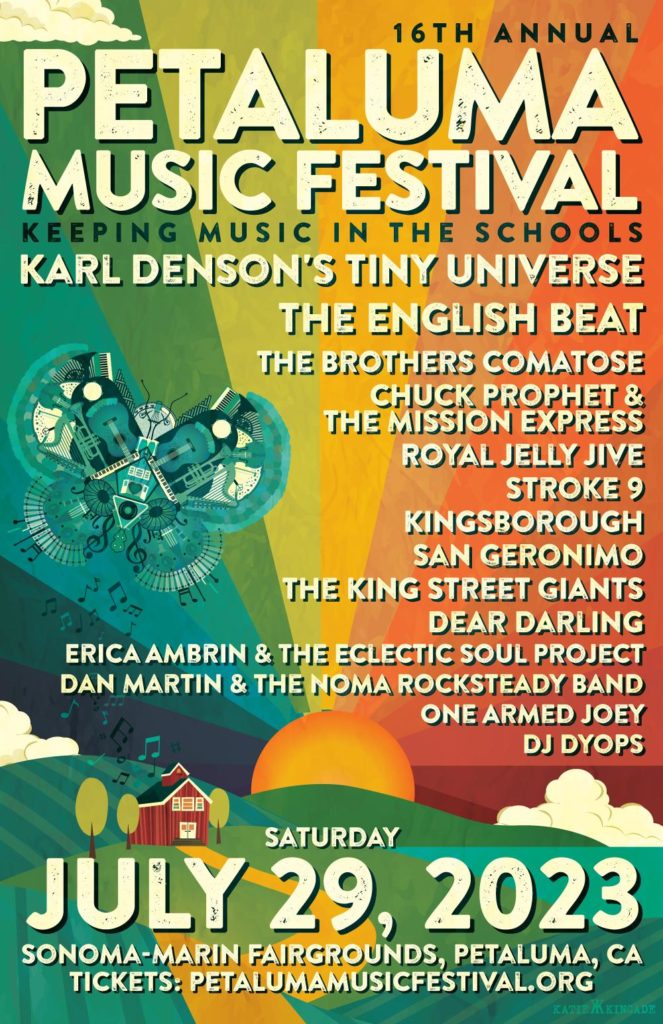**Poster Description:**

The digital poster captures a vibrant and scenic sunrise, evoking the spirit of a summer music festival. The background features a pristine hillside adorned in varying shades of green, highlighted with stripes of deeper green, and split by a winding yellow road that meanders through the landscape. Rising from behind the hill, an orange sun casts its radiant, rainbow-colored rays across the sky. The left side of the sun's rays transitions through shades of red and pink, while the middle hues move from yellow to green, and the right side shifts from light blue to purple.

Prominently displayed in white text, the poster announces the "16th Annual Petaluma Music Festival," with a special emphasis on "keeping music in the schools" in larger, standout type. Below this, a roster of featured bands includes:

- Carl Denson's Tiny Universe
- The English Beat
- The Brothers Comatose
- Chuck Prophet & The Mission Express
- Royal Jelly Jive
- Stroke 9
- Kingsborough
- San Geronimo
- The King Street Giants
- Dear Darling
- Erica Ambrin & the Eclectic Soul Project
- Dan Martin & The Noma Rock Steady Band
- One Arm Joey
- DJ Deops

The festival is set to take place on Saturday, July 29th, 2023, at the Sonoma-Marin Fairgrounds in Petaluma, California. More details and ticket information can be found at petalumamusicfestival.org. Notably, the text "16th annual" and "keeping music in the schools" stands out, highlighted in a contrasting color to draw attention.